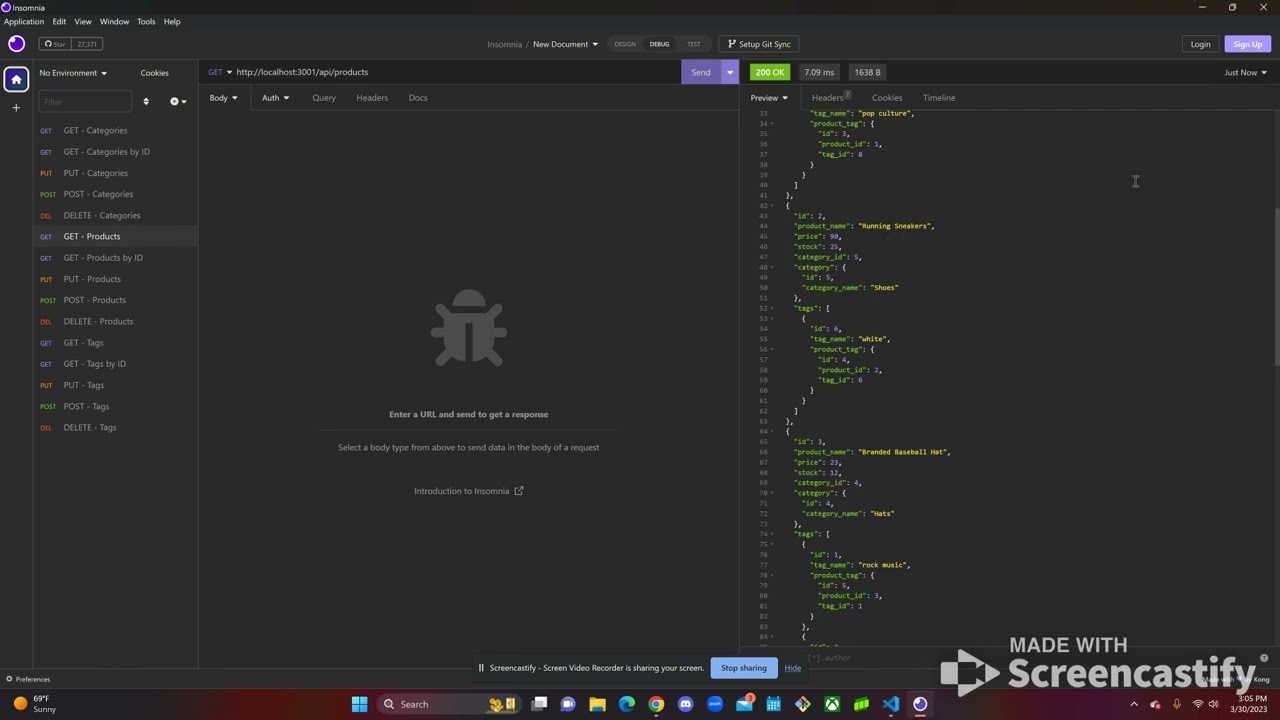This image is a detailed screenshot of a Windows computer screen displaying a webpage or an application with a black background, possibly related to coding. The bottom right corner prominently features the Screencastify logo and watermark. Across the bottom bar of the screen, various icons are visible, indicating open applications such as Google Chrome, Xbox, Mail, Calendar, Internet Explorer, and more. 

The screen is divided into several sections: 
1. **Top Navigation Bar**: This bar includes options for Application, Edit, View, Window, Tools, and Help, along with buttons for logging in and signing up in the upper right corner.
2. **Left Sidebar**: This sidebar contains a list of options in white and orange text, prompting the user to enter a URL.
3. **Main Panel**: The centerpiece of the screen features an image of a gray bug, which resembles a ladybug, adjacent to some white text.
4. **Right Panel**: This section displays what appears to be HTML code, with rows numbered in white and code highlighted in green and yellow. 

Additional information includes the date, time, weather (sunny), and system icons for microphone and Wi-Fi in the lower right corner, confirming the user is on a Windows operating system.